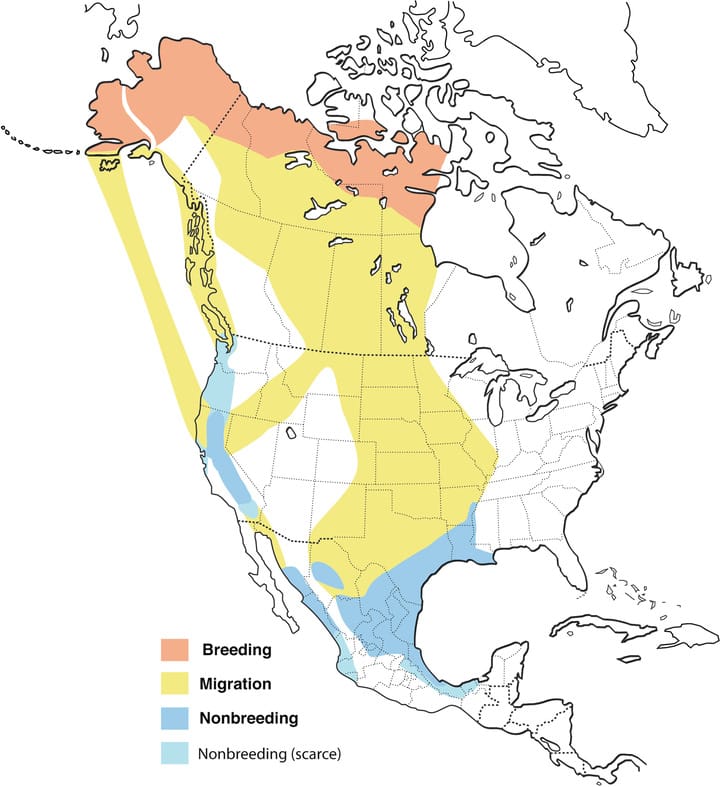The image is a detailed map of North America including Canada, the United States, and Mexico, accompanied by a color-coded key on the bottom left designating different regions based on bird activity. The key includes four colors: orange for breeding, yellow for migration, dark blue for non-breeding, and light blue for scarce non-breeding. Most of the map is marked yellow, indicating areas of migration, extending from central Canada down through the central United States and areas towards California. A small patch of orange, indicating breeding, is visible in the northernmost parts of Canada and reaches slightly into Alaska. Dark blue sections, indicating non-breeding areas, appear along the west coast from California down into Mexico, with an additional patch in Mexico extending to the northeast towards Texas and Louisiana. Light blue areas, representing scarce non-breeding locations, are found on the borders of these dark blue sections. The rest of North America, including the eastern United States from Florida to Louisiana, Alabama, Michigan, Ohio, and into parts of Canada, remains uncolored, marked as white.